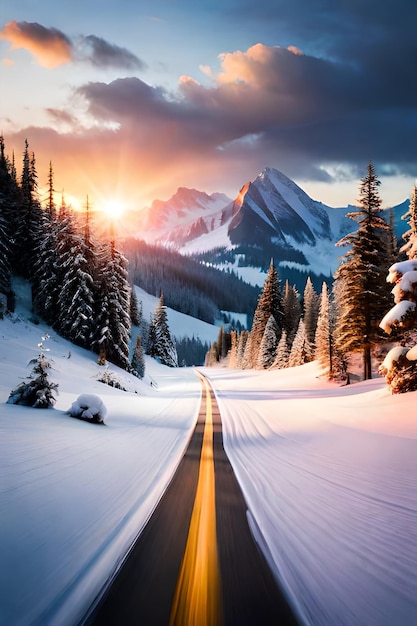The image depicts a serene winter landscape captured digitally in a vertical frame. Central to the composition is a snow-dusted black asphalt road, marked with a prominent yellow line, that extends from the viewer's perspective into the middle distance. On either side of the road lies a blanket of snow, giving way to snowy fields and clusters of towering coniferous trees. The trees are mostly green, though some branches, particularly on the left side of the image, glisten with snow. Beyond the road and trees, the eye is drawn to two distant, majestic, snow-covered mountains. A delicate pinkish hue graces one of the mountain peaks, illuminated by the faint sun peeking just above them. The sky, adorned with dark clouds, is predominantly blue and suggests either a sunset or sunrise, casting a warm glow over the entire scene. This juxtaposition of the dark clouds and vibrant sky, combined with the soft glare from the sun, creates a compelling contrast and a tranquil atmosphere.